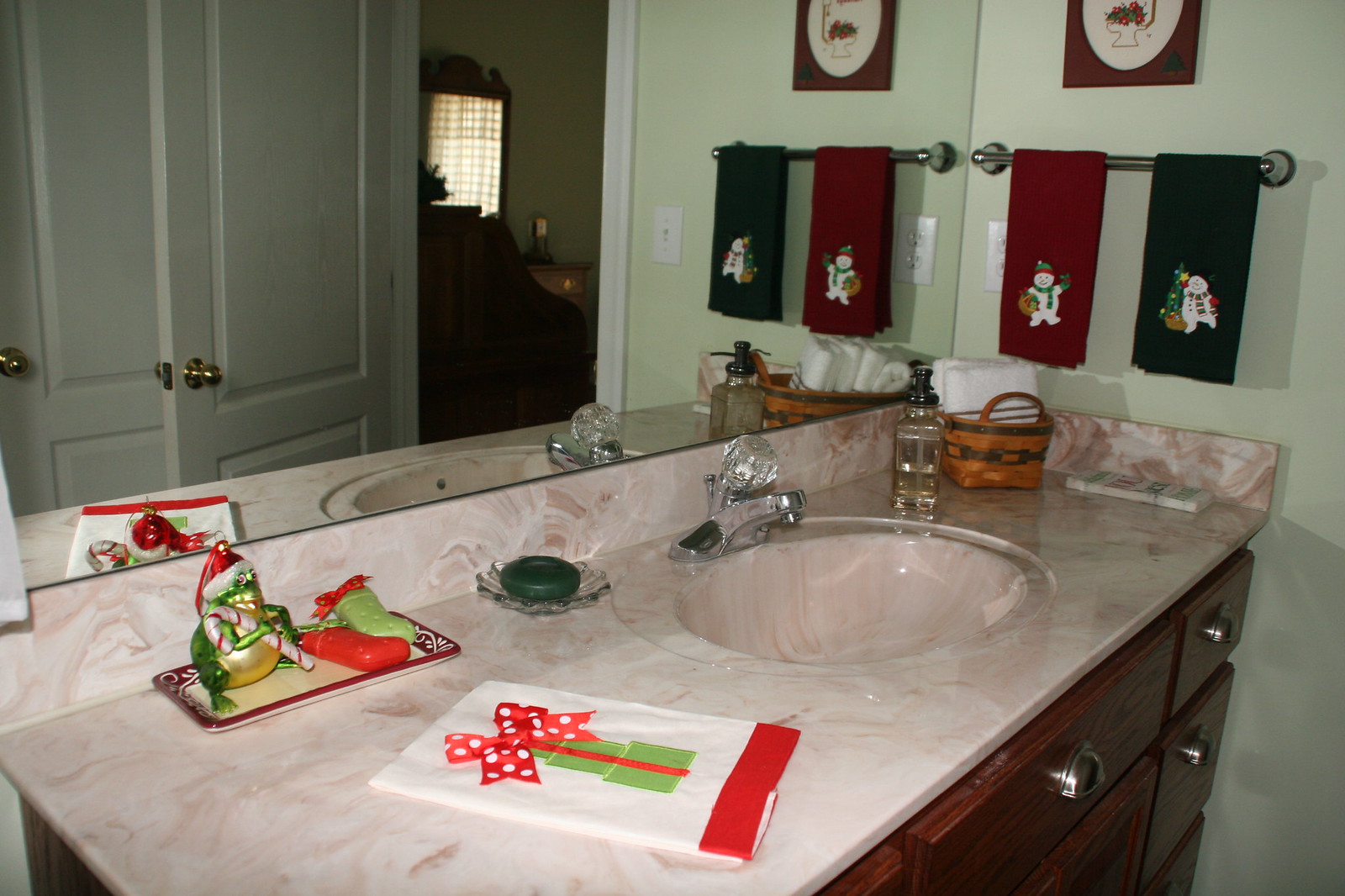A festive, well-lit photo showcases a Christmas-themed bathroom counter. The countertop is made of creamy marble, giving it a luxurious feel, and is supported by dark wood drawers adorned with sleek, silver handles. A large mirror on the left dominates the wall, reflecting an adjacent open doorway leading to another room and a closed door. Hanging from a towel rack in the background are two vibrant towels: one red and one green, each featuring embroidered snowmen in festive scarves and hats. An additional needlepoint item, whose image is indiscernible, is hung above the towels. 

In the foreground, a white towel with a red border and bow is neatly folded next to a small green box, creating the look of a wrapped present. Underneath the mirror, a frog figurine sporting a Santa hat adds a whimsical touch. Nearby, a small glass dish holds a cutesy bar of green soap. The single sink is flanked by a clear plastic pump bottle and a wooden basket filled with neatly folded towels. At the far end of the counter, an unidentified item rests against the wall, completing the festive Christmas decor.